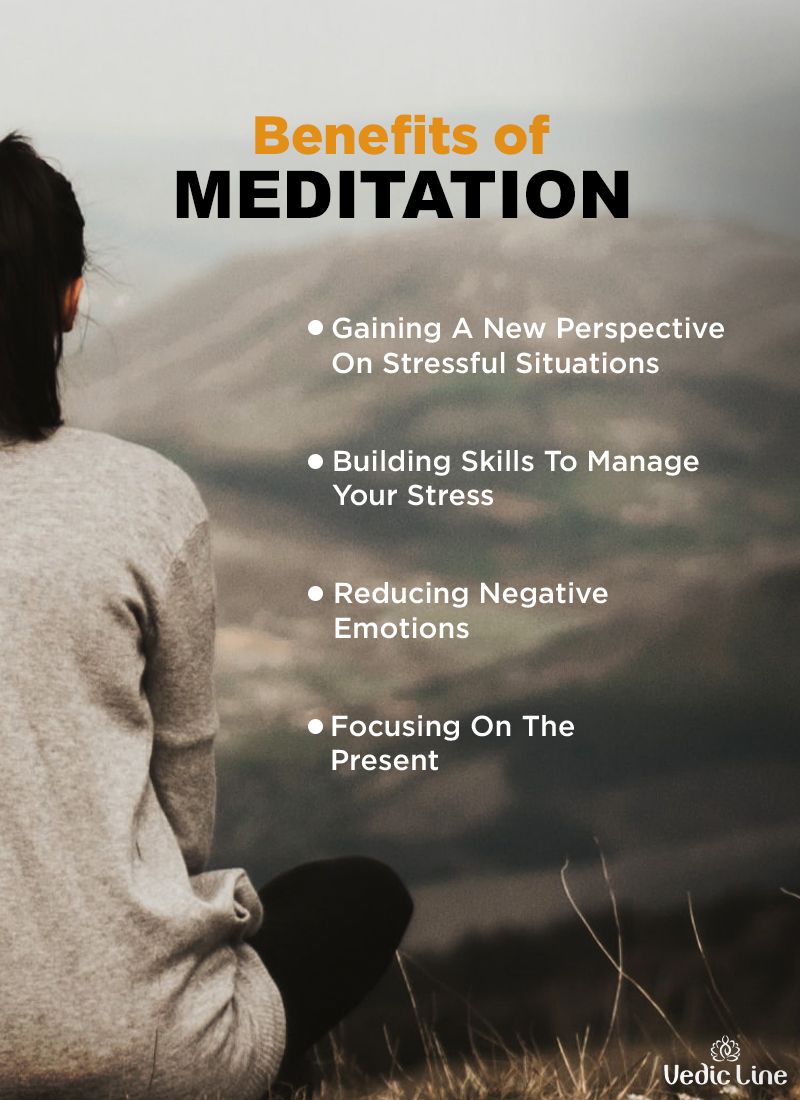The image is a rectangular, possibly poster-like graphic, predominantly featuring a serene scene intended for a self-help or meditation promotional material. Central to the image is a woman with dark hair, wearing a gray long-sleeved shirt and black leggings, sitting cross-legged on yellowing grass indicative of early spring or fall. She faces away from the camera, gazing into the distance towards a blurred, tranquil landscape that includes mountains and possibly a river valley, all under a gray sky.

The primary focus is on the text overlaying the upper portion of the photograph, with the title "Benefits of Meditation" in orange, followed by four key points in white text: "Gaining a New Perspective on Stressful Situations," "Building Skills to Manage Your Stress," "Reducing Negative Emotions," and "Focusing on the Present." The bottom right corner of the graphic features the brand name "VedicLine" accompanied by an indiscernible small symbol above it, both in white text. The overall ambiance of the image is calming and zen-like, emphasized by wisps of grass around the woman and the foggy, distant mountains.